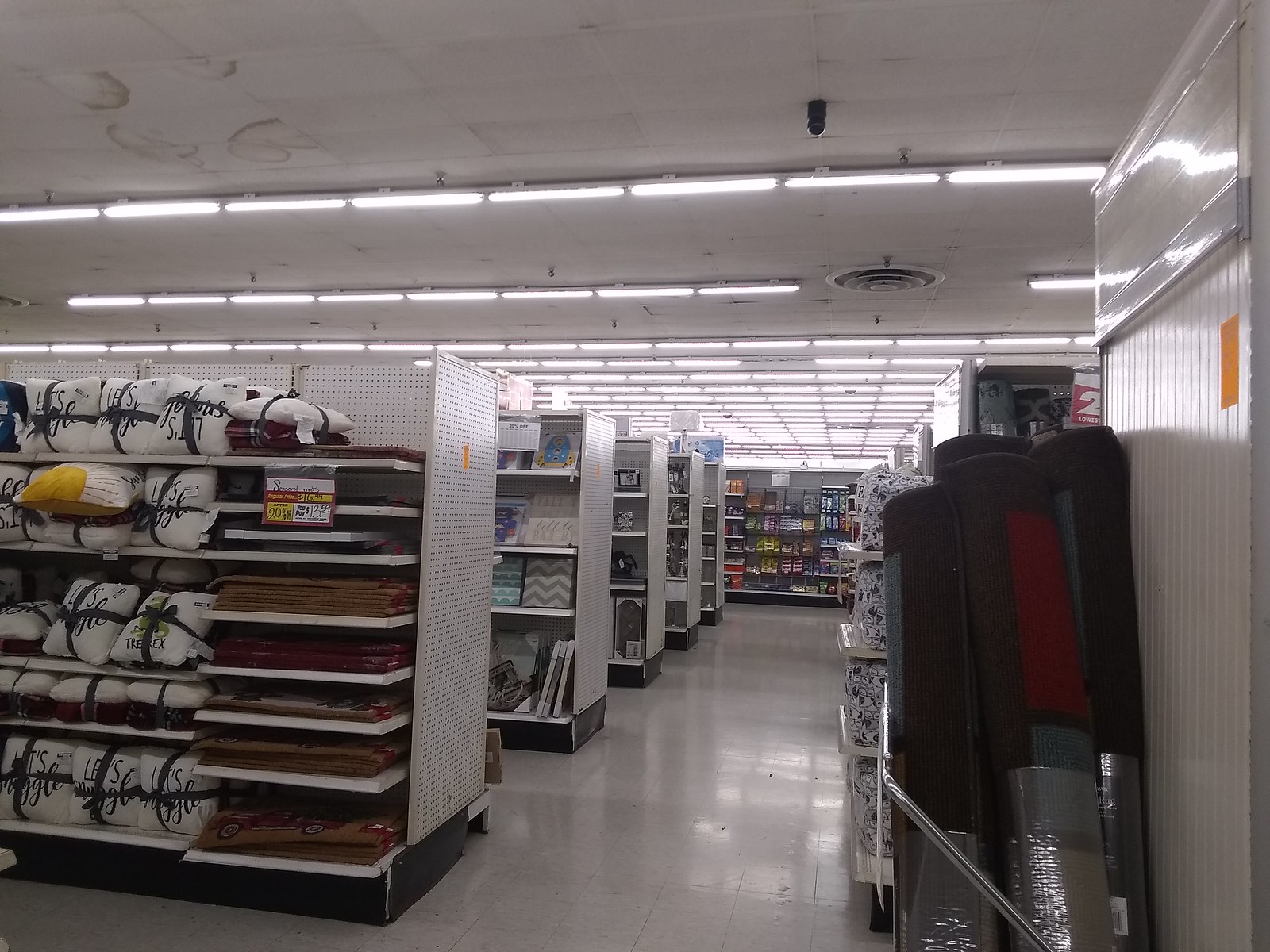This photo captures the interior of a retail store, devoid of customers, showcasing a quiet, organized shopping environment. The focus is on one side of the store, where the left features several aisles lined with merchandise. In the immediate foreground, an aisle is stocked with throw pillows neatly arranged on multiple shelves, each shelf appearing to hold identical pillows. Adjacent to this aisle, on the end cap, a flat item, likely a welcome mat, is displayed. Moving further down, the next row displays wall plaques adorned with inspirational sayings. Beyond these, additional aisles, whose contents remain unspecified, extend towards the back of the store. 

Directly ahead, a gray wall comes into view, outfitted with several black shelves laden with various items for sale. On the right side of the image, a white wall holds several large rolled-up carpet pieces or area rugs, leaning against it in tidy rows. 

The store's floor is covered in white linoleum, providing a clean and bright surface, while the ceiling is lined with tiled panels interspersed with fluorescent light tracks, ensuring the space is well-lit throughout.